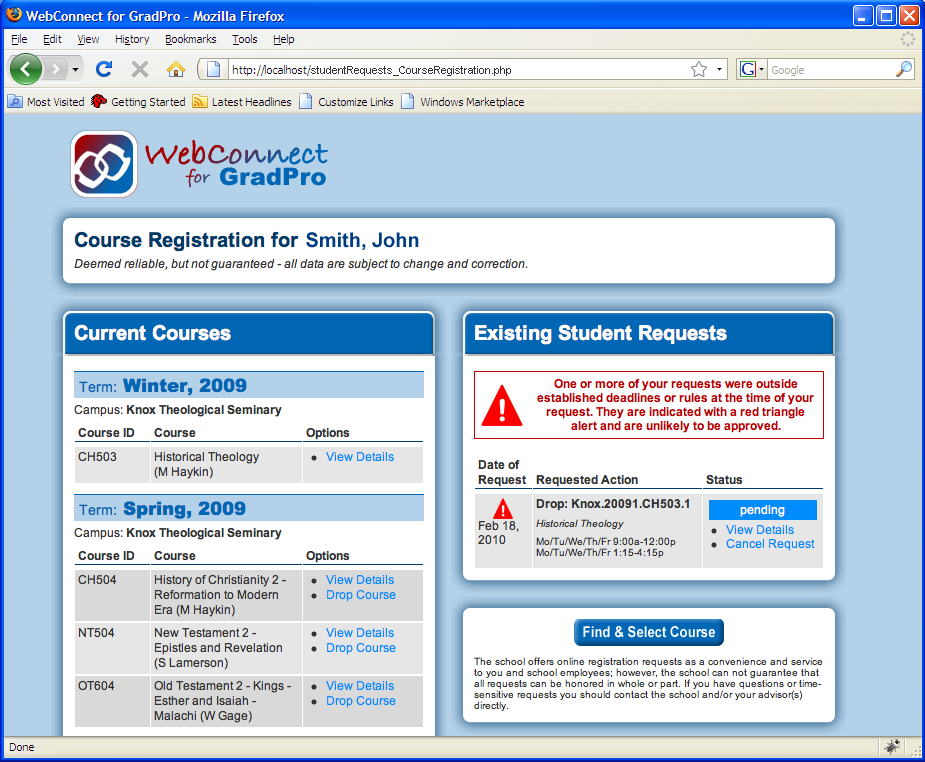This image depicts a webpage displayed within the Mozilla Firefox browser. At the top of the screen, there is a blue banner featuring the Firefox logo in the upper-left corner. Beside the logo, white text reads "WebConnect for GradPro - Mozilla Firefox," with "WebConnect" and "GradPro" displayed as single words, each capitalizing the letters "W" and "C" for WebConnect and "G" and "P" for GradPro.

To the upper-right, standard browser window controls are visible: an "X" button to close the window, a line icon to minimize it, and a square icon to maximize it. Below the blue banner is a navigation bar with menu options including File, Edit, View, History, Bookmarks, Tools, and Help.

Directly beneath this navigation bar, there are standard browser navigation controls: a back arrow housed in a circular icon, a grayed-out forward arrow, a blue refresh button, an "X" to stop loading, a home icon, an address bar containing the website URL, followed by a separate search bar.

The main content of the webpage is divided into several sections. Below the browser controls, there is a row of links labeled "Most Visited," "Getting Started," "Latest Headlines," "Customized Links," and "Windows Marketplace." The background primarily appears in blue hues.

Central to the page’s main area is a rounded square icon with an image resembling handcuffs, next to the text "WebConnect for GradPro." Beneath that, a white banner reads "Course Registration" and further details, displaying "Course Registration for Smith, John."

The page then lists "Current Courses" followed by terms, notably "Winter" and "Spring 2009," with sections for "Existing Student Requests," "Final" and "Selected Courses," clearly laid out in structured lists.